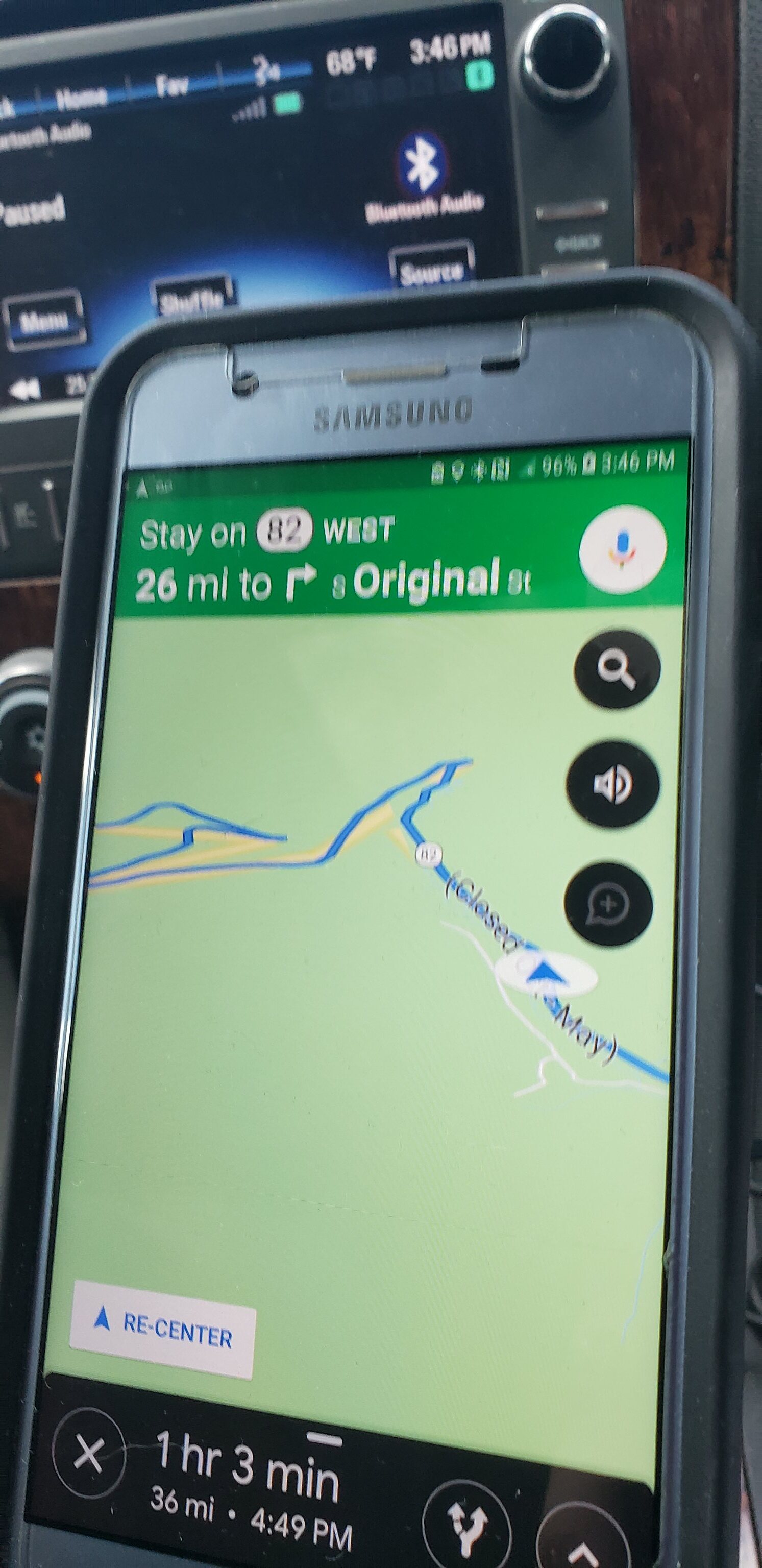The image captures a Samsung smartphone, prominently featuring a black case, mounted in a vehicle giving navigation directions. The phone's screen displays a map application with detailed guidance, including a blue route line on 82 West highlighted with a current location marker. It instructs the user to stay on 82 West for 26 miles before making a right turn on South Original Street. The navigation banner at the top is in white writing on a green background. At the bottom, key trip information is noted: "one hour three minutes, 36 miles" and an estimated arrival time of 4:49 p.m. The background shows part of the car's dashboard, which includes a smart screen showing paused Bluetooth audio, and several control buttons and dials labeled “menu,” “shuffle,” and “source.” Some side panels appear to have a grayish chrome finish, adding a sleek look to the vehicle's interior.